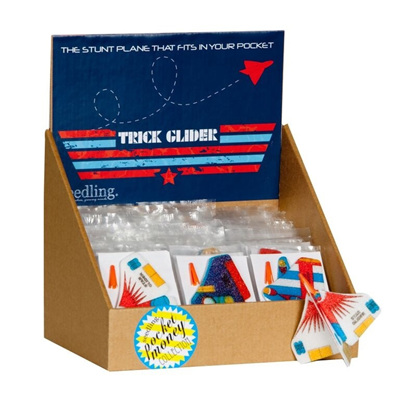The image depicts a light brown toy compartment filled with approximately twenty "Trick-O-Lighter" toys, organized across multiple levels. The compartment is set against a white backdrop, and prominently displays a pop-up sign with the logo "Trick-O-Lighter" in red, blue, and white. Above the logo, a red plane with a dotted line trails off to the right, accompanied by the slogan "The stunt plane that fits in your pocket." The display showcases one of the unwrapped "Trick-O-Lighter" toys at the front, revealing its flat wings and horizontal middle section, resembling a mini stunt plane. Additionally, a sticker on the front of the compartment reads "Pocket Money Collection" in yellow, white, and blue.